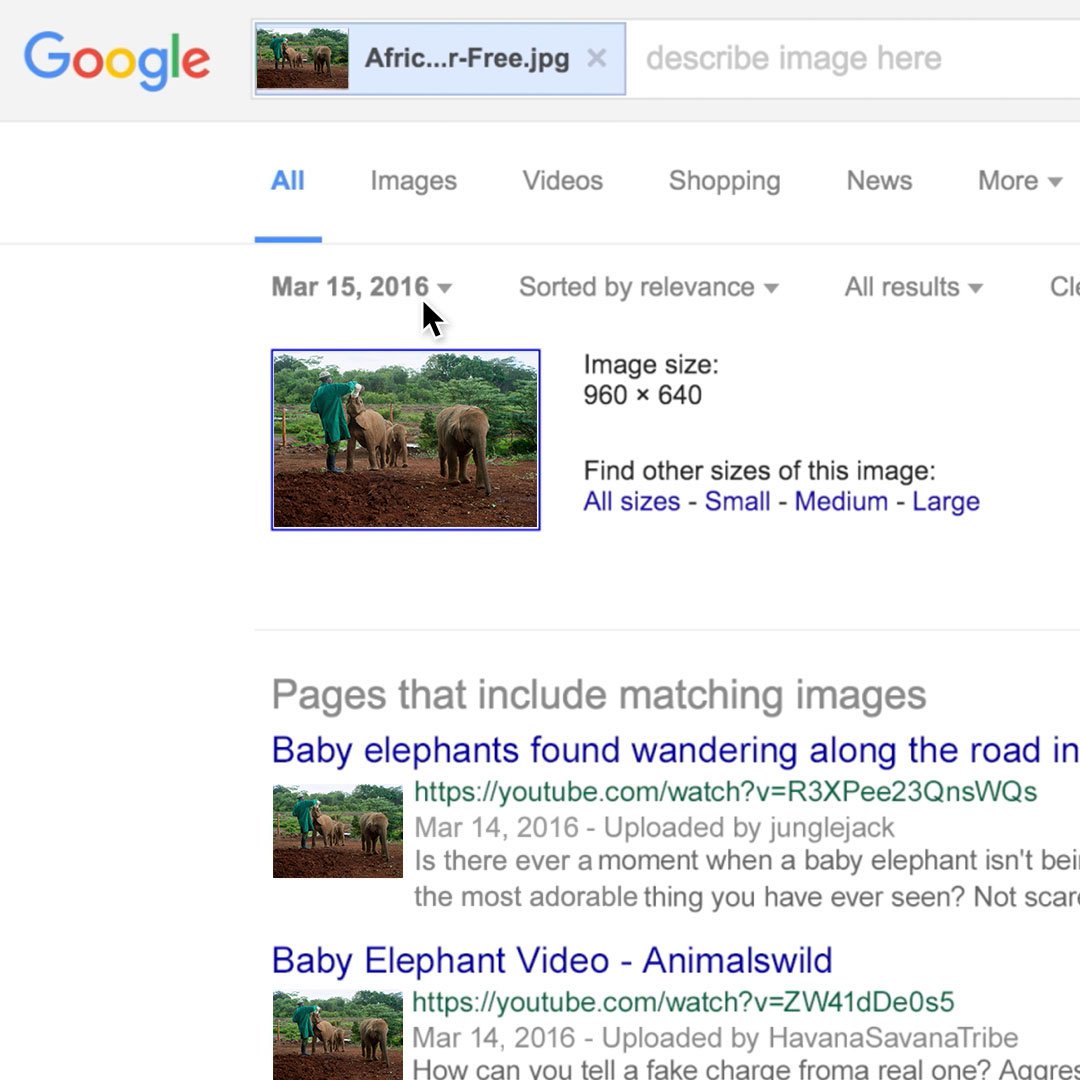The image displays a Google search results page with a query for "Africa free dot JPEG." At the top of the page, the traditional Google logo is prominently featured in its recognizable multicolored scheme: blue 'G,' red 'O,' yellow 'O,' blue 'G,' green 'L,' and red 'E.' Below the logo, the search box contains the entered query. 

The interface presents various categories including "All," "Images," "Videos," "Shopping," "News," and "More," alongside additional filtering options like "Sort by relevance" and a timestamp dated "March 15th, 2016." The search results indicate an available image with dimensions of 960 by 640 pixels, offering the choice to find other sizes categorized as small, medium, and large.

The featured image portrays a heartwarming scene of two smaller elephants standing beside a person wearing a green jacket and a hat who appears to be feeding them. Accompanying the visual is the text: "Pages that include matching images: Baby elephants found wandering along the road in," followed by the hint of an incomplete sentence. The page further includes a link to a baby elephant video titled "Animals wild," dated March 14th, 2016, and uploaded by the Havana Savannah tribe. Finally, there's a thought-provoking question: "How can you tell a fake charge from a real one?"